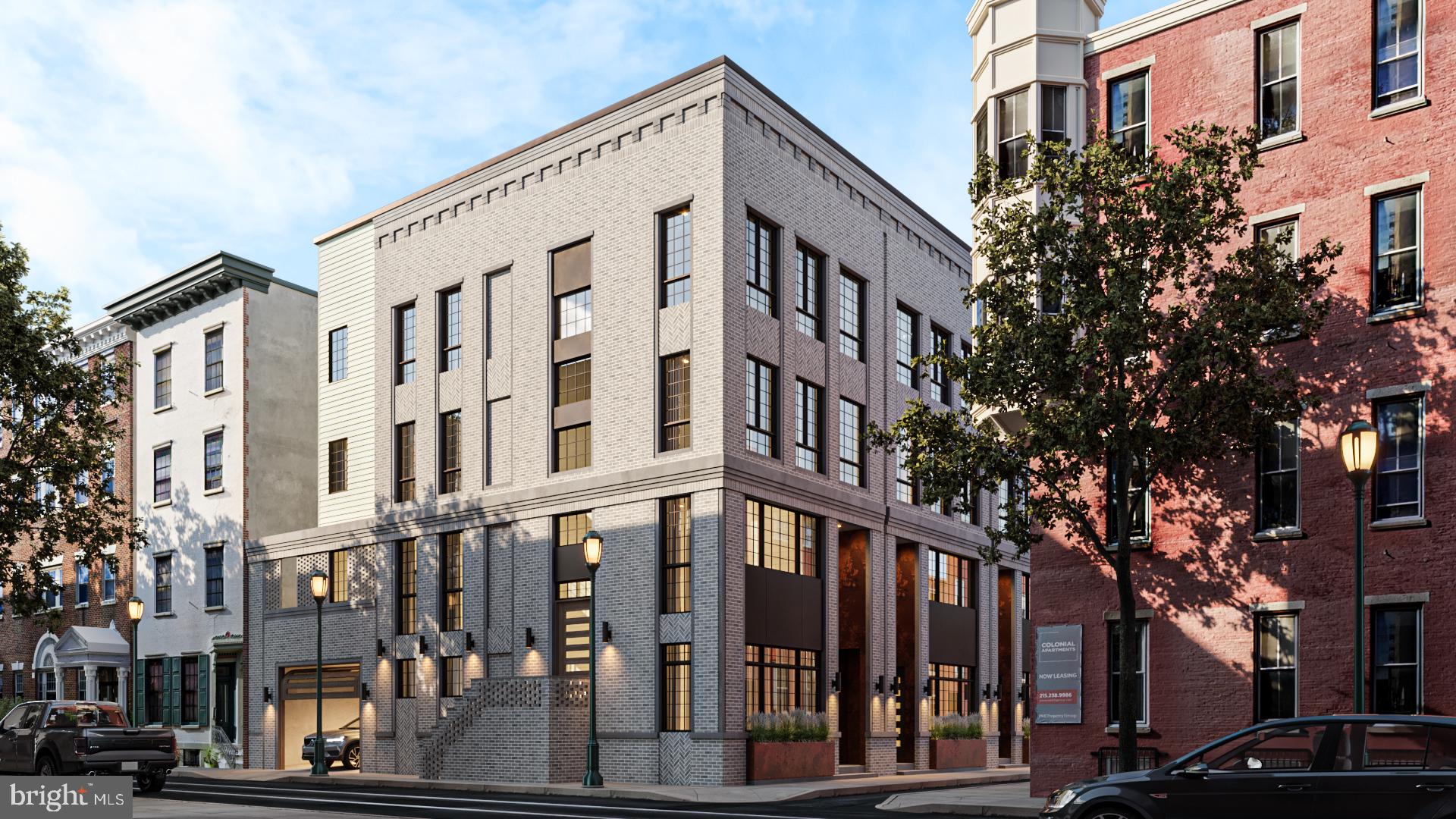The image showcases a city block with a set of buildings and a street. The primary focus is on a white concrete building on the corner, featuring a two-story shop on the ground floor and additional stories above with rows of windows. Adjacent to this, a second white building, likely an apartment complex, rises four stories high. To the right, a red brick building also stands four stories tall, partially obscured by a tree in front. The red brick building sits near an alley and a small parking area, where a car is visible. There is also a ladder or staircase structure extending from the front of one of the buildings. The sky above is mostly clear with patches of white clouds. Furthermore, the image includes an overlay text reading "bright MLS," and multiple streetlamps are present along the sidewalk. The overall setting imparts a small, old-town business district atmosphere.